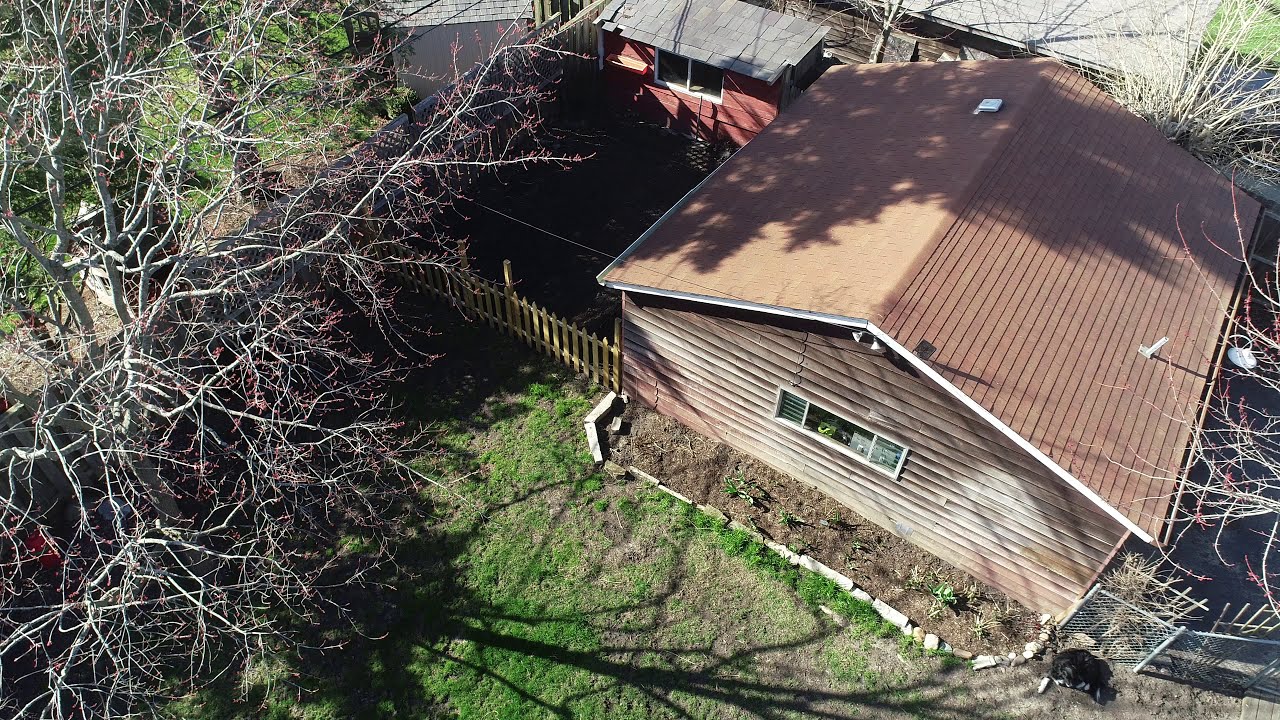This aerial photograph captures a quaint, small family house situated on the right side of the image, with a distinctive brown A-frame, tiled roof. The house, constructed from horizontal wooden slats that have weathered over time to a dark, faded brown, is single-story and features a central horizontal window. The bottom part of the image reveals the back of the house with a modest garden outlined by stones, mostly consisting of dirt. Flanking the house's left, a tall, barren tree extends its leafless branches towards the viewer, dominating the left-hand side of the frame. Adjacent to the house on the right, a green grassy yard stretches out, interrupted by a small wooden gate and another area presumed to be a driveway. In the backyard near the right side gate, an animal, possibly a dog, lies peacefully. Additionally, there is a small red shed with a gray roof to the left side, next to a cement area, providing a structural balance to the scene. Beyond the house, the boundaries fade into more surrounding trees, their skeletal branches further framing this serene and rustic setting.